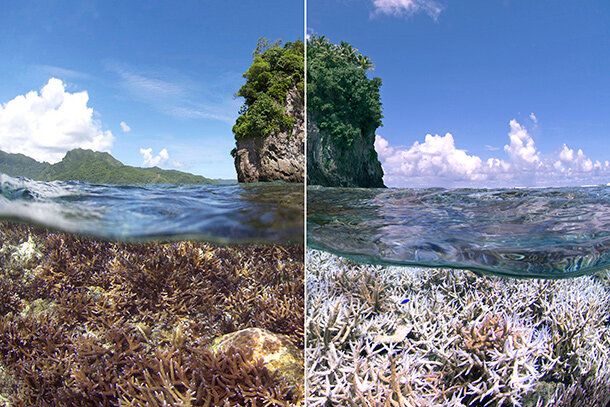The combined photograph showcases a striking before-and-after comparison of a coastal landscape. The two sections of the image are divided by a white line, with the left side portraying a vibrant, pristine environment, and the right side revealing noticeable ecological decay. Dominating the center of both halves is a towering rock formation, adorned with green foliage and trees. The sky above is a brilliant cyan blue, dotted with white, billowy clouds.

On the left, the scenery is lush and alive; green mountains rise in the background, covered in dense foliage, and the crystal-clear water below reveals thriving brown and orange coral interspersed with yellow and beige hues. The sunlight bathes the scene, emphasizing the clarity and vivid colors.

In contrast, the right side displays a darker, more somber atmosphere. The formerly green-clad mountains are veiled in multiple clouds, and the predominant foliage on the cliff has grown denser and darker in color. Beneath the surface, the once-vibrant coral has faded to a pale beige, signifying its death. Although the day remains bright with similar clear skies, the water appears slightly ripply but still calm, adding to the haunting transformation depicted between the two halves of the photograph.